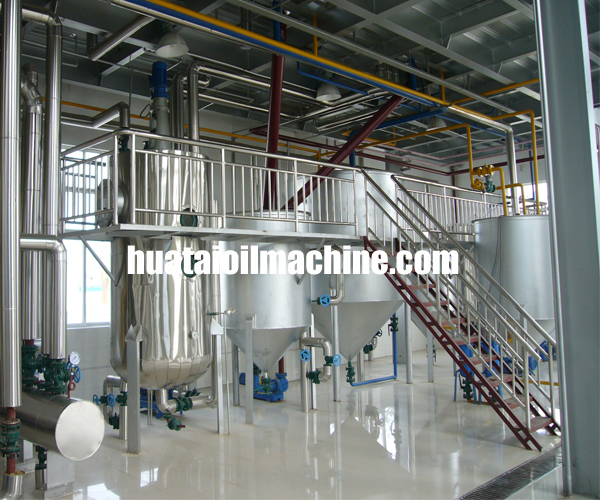The image depicts the interior of a factory, characterized by its industrial layout and machinery. Prominent in the background are several large silver drums, which taper to a point at the bottom and feature blue accents. These drums are likely storage units for some type of oil, as suggested by the superimposed white text in the middle of the image that reads "HUATAI OIL MACHINE.COM".

The factory floor is exceptionally clean and shiny, with a white hue that reflects the surrounding equipment. The walls also appear white, while the ceiling contrasts with a gray tone. 

A steel beam anchors the right side of the composition, adding to the robust industrial aesthetic. Numerous pipes, including notable gold ones running along the ceiling and additional pipes clustered on the left, interconnect the machinery, facilitating the movement of materials throughout the facility. Several levers are visible among the pipes, probably used to control the flow.

In the center, a metal staircase ascends to a catwalk or second-story platform equipped with a guardrail, potentially used by workers to access the tops of the vats for maintenance or monitoring tasks. The overall scene conveys a highly organized and well-maintained industrial environment geared towards oil processing.